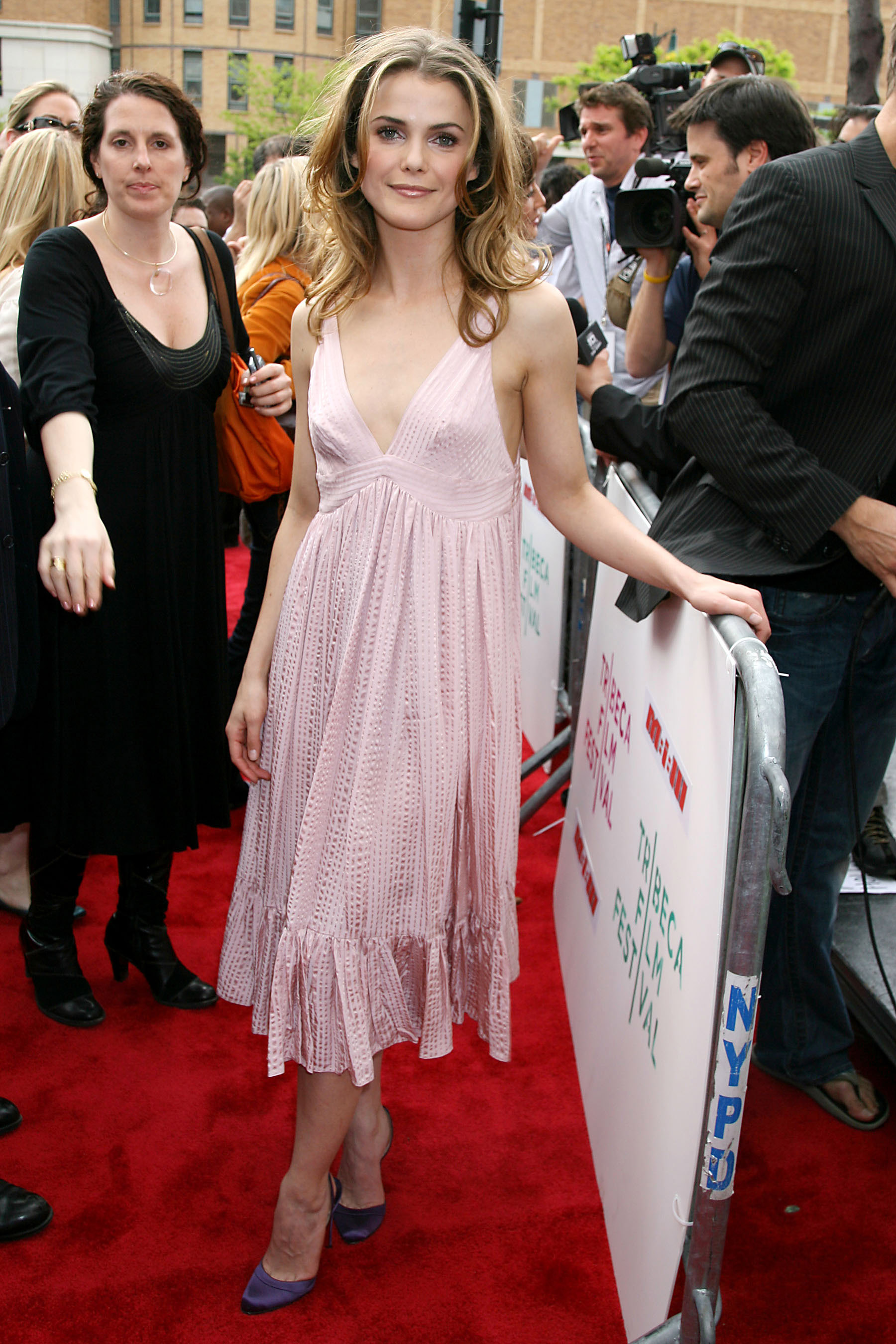The photograph depicts Keri Russell, a white female actress, standing at the center of a bustling red carpet event during the Tribeca Film Festival. She is wearing a pastel pink spaghetti-strapped dress featuring a low V-neck cut and is complemented by striking purple high-heeled pumps. Her shoulder-length, brownish-blonde hair cascades gently around her face as she leans against a sign that reads "Tribeca Film Festival," gazing directly at the camera. The scene is vibrant and busy, with well-dressed photographers, news reporters, and a general crowd visible in the background, some holding microphones and cameras. The setting is outdoors in daylight, framed by distant buildings and trees, adding to the lively and glamorous atmosphere of the film festival. Her left hand rests on a metal grating fence, partially obscuring a white square with unreadable text. The dominant colors in the scene include shades of red, pink, tan, black, green, blue, and gray, enhancing the vividness of the moment captured.